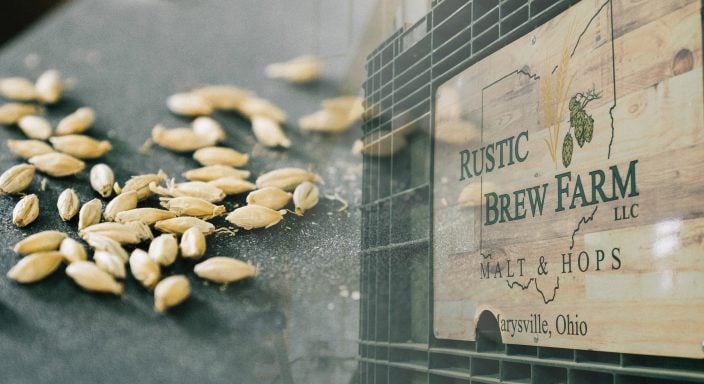The image is a horizontally oriented, rectangular photograph featuring a prominent wooden sign with green lettering that reads "Rustic Brew Farm LLC," followed by "Malt and Hops, Marysville, Ohio." The background also displays a map outline of Ohio with green plant imagery and yellow wheat, emphasizing the farm's local heritage. In the foreground, on the left side of the image, there is a small pile of around 15 to 30 beige, pellet-like hops scattered across a gray table with white specks. A green basket or crate partially filled with these hops is visible on the right side, complementing the rustic, farm-themed aesthetic. The detailed setting creates a visually rich marketing image for Rustic Brew Farm.